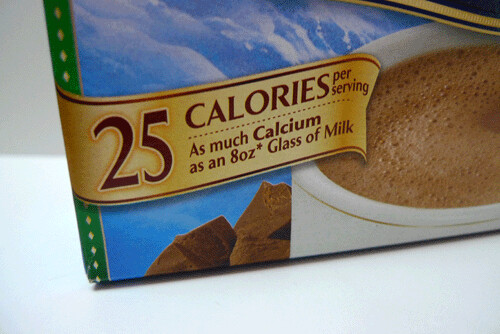The image depicts the bottom left corner of a box of hot chocolate mix resting on a white surface. The box features a captivating scene on its front side, with a vivid blue sky and fluffy white clouds in the background. Prominently displayed is a white coffee mug filled with hot chocolate, characterized by a frothy, bubbly top. Next to the mug are several chunks of broken dark brown chocolate. A gold banner wraps around from the side to the front of the box, embossed with black letters stating, "25 calories per serving. As much calcium as an 8-ounce glass of milk." The side of the box is green with a series of white dots running along its edge, adding a touch of contrast to the packaging.